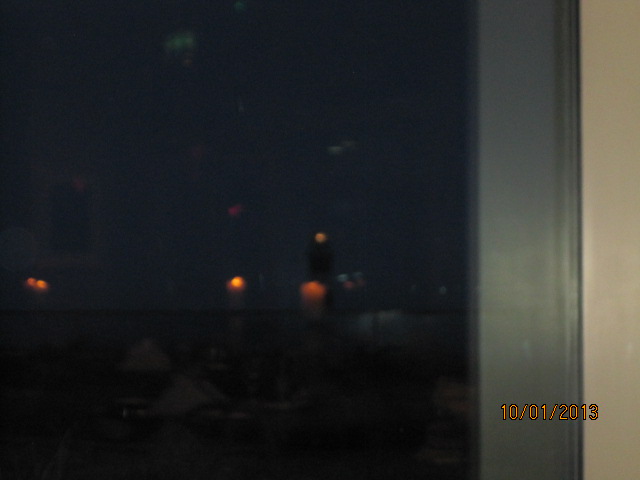The image is a low-quality, low-resolution, blurry square photograph. The overall image is quite fuzzy, making it difficult to discern specific details. On the bottom right corner, an orange-colored text reads "10-101-202013." The right side of the image features a white section, while the left side is dominated by a dark teal-colored area. The majority of the image remains indistinct and unclear, reflecting its poor quality.